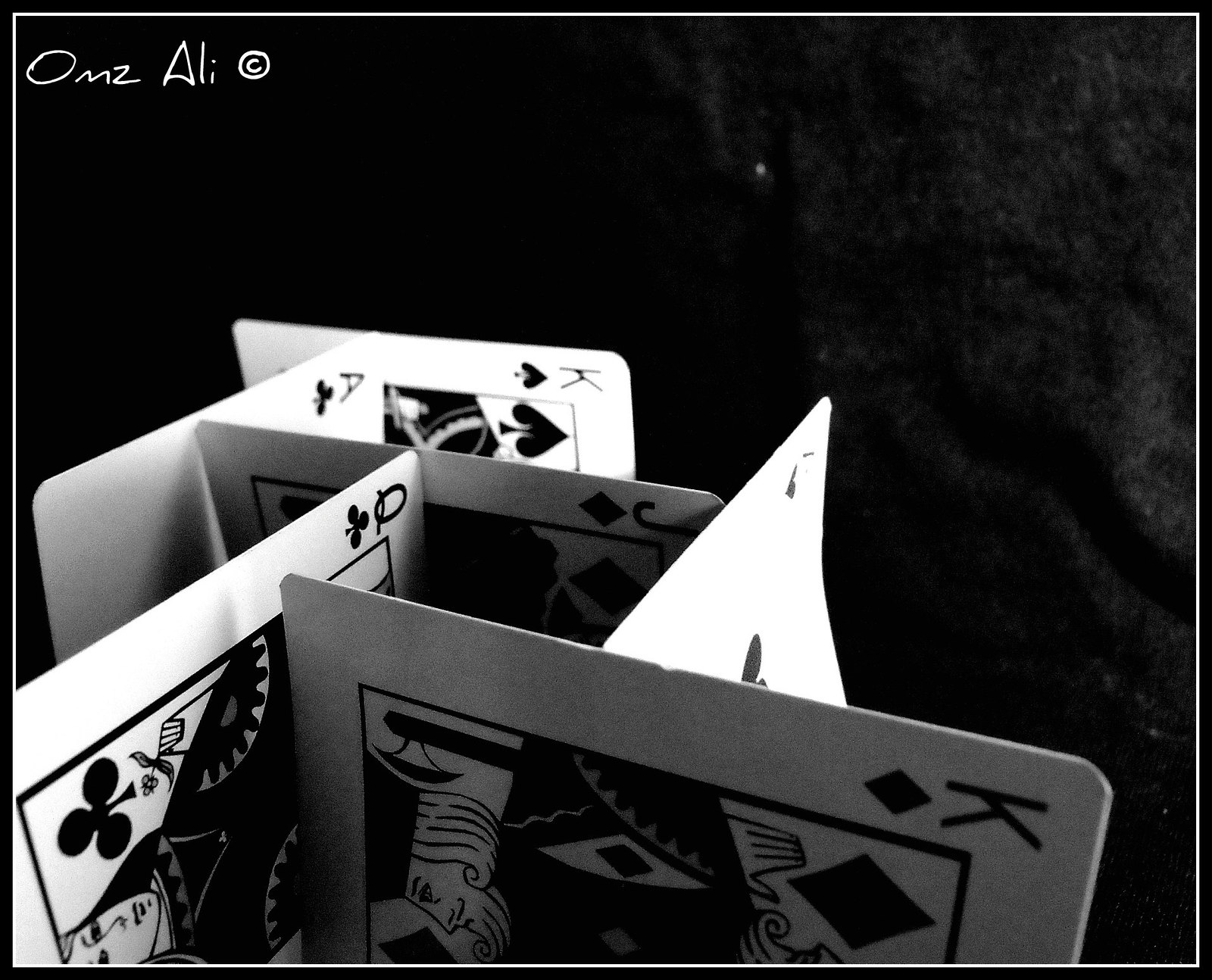The image features a close-up view of six playing cards meticulously arranged against a black fabric backdrop. The photograph is framed with a thin white border, followed by a thicker black border, enhancing its sleek and dramatic composition. In the top left corner, "OMZALI copyright" is inscribed in white text, accrediting the creator.

The cards are set upright and slightly tilted, creating a visually engaging, cascading pattern where each card seems to be delicately leaning against its neighbor. The foremost card is the King of Diamonds, exhibiting the traditional dual image of the king, with one facing left and the other right. Propped against the King of Diamonds, the Two of Hearts tilts upward toward the top right corner.

Adjacent to this, a Queen of Clubs aligns with the King of Diamonds, adding to the intricate arrangement. Behind these cards, the Jack of Diamonds is subtly angled downward to the left, and above it, the Ace of Clubs stands prominently. The farthest card in the arrangement is the King of Spades, completing the set.

The entire image is rendered in black and white, stripping the cards of their usual colors and lending a timeless, elegant quality to the scene.